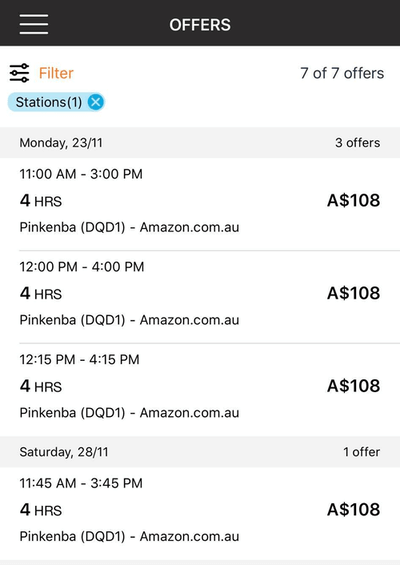The screenshot depicts a mobile phone interface featuring a black top banner with a white "hamburger" menu icon on the left and the word "OFFERS" in bold, all-caps text at the center. Below the banner, there is a "FILTER" icon that allows users to filter the offers displayed. 

The main content area shows that there are 7 offers available from a station, and it allows users to exit the view if desired. The offers are listed with specific details:

1. **Monday, November 23**:
   - **Time**: 11:00 AM to 3:00 PM
   - **Duration**: 4 hours
   - **Cost**: AUD 108
   - **Location**: Pinkabah
   - **Vendor**: Amazon.com.au

2. **Another offer on the same day**:
   - **Time**: 12:00 PM to 4:00 PM
   - **Duration**: 4 hours
   - **Cost**: AUD 108
   - **Location**: Pinkabah
   - **Vendor**: Amazon.com.au

3. **Third offer on the same day**:
   - **Time**: 12:15 PM to 4:15 PM
   - **Duration**: 4 hours
   - **Cost**: AUD 108
   - **Location**: Pinkabah
   - **Vendor**: Amazon.com.au

4. **Saturday, November 28**:
   - **Time**: 11:45 AM to 3:45 PM
   - **Duration**: 4 hours
   - **Cost**: AUD 108
   - **Location**: Pinkabah
   - **Vendor**: Amazon.com.au

The interface indicates that the user is viewing 7 out of 7 offers, and additional details can be seen by scrolling down. The offers are identical in terms of cost and duration, but vary by specific times, allowing the user to choose according to their availability.